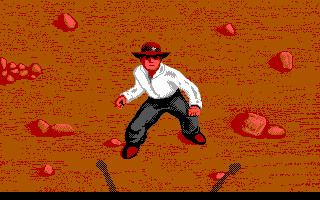This image, likely a screenshot from a video game, features a cowboyish character standing in its center. The character, who resembles Indiana Jones, sports a brown cowboy hat adorned with a black band and a silver insignia, a long-sleeved white shirt, black pants, and brown boots. His face, turned towards the viewer, clearly shows his eyes, nose, and mouth. His right hand is bent back as if ready to throw something, while both fists are somewhat balled up. The background is a deeper brown color dotted with red, with red stones scattered across the ground, suggesting a desert-like environment. Additionally, the image has a distinctive black line at the bottom extending from left to right, with two gray lines diverging from it and pointing towards the upper left and upper right corners.